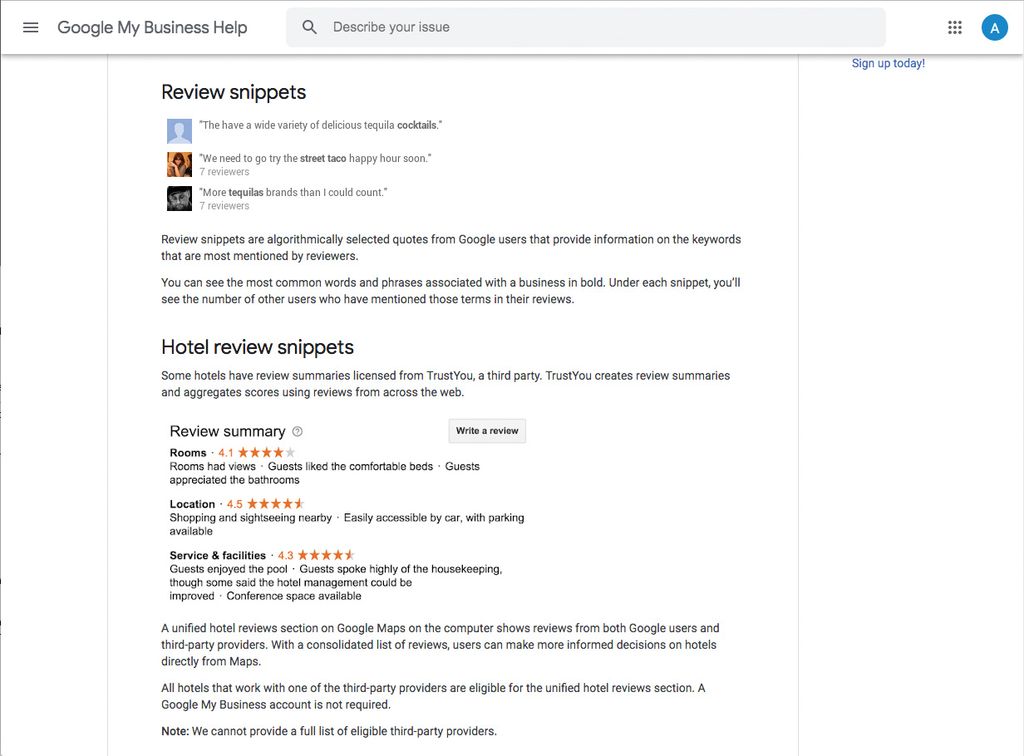This is an image of the "Google My Business Help" website interface. On the left sidebar, the title reads "Google My Business Help," and in the central browsing area, there's a prominent gray search bar labeled "Describe your issue." Below the search bar, there are three vertically aligned icons: the top icon is blue, the middle one is a combination of orange and blue and appears to represent a real person, and the bottom one has an image within a black box.

To the right of the icons, there's a text block explaining review snippets. The text states: "Our review snippets are algorithmically selected quotes from Google users that provide information on the keywords that are most mentioned by reviewers."

In the central part of the screen, the section titled "Hotel Review Snippets" details that some hotel reviews are summarized by a third-party service called TrustYou, which aggregates scores and creates review summaries from reviews across the web. There is a review summary section showing star ratings for various categories such as rooms, location, service, and facilities, with stars depicting the rating for each category. Below this, two paragraphs discuss hotel reviews in detail. The section ends with a note stating: "Note: We cannot provide a full list of eligible third-party providers."